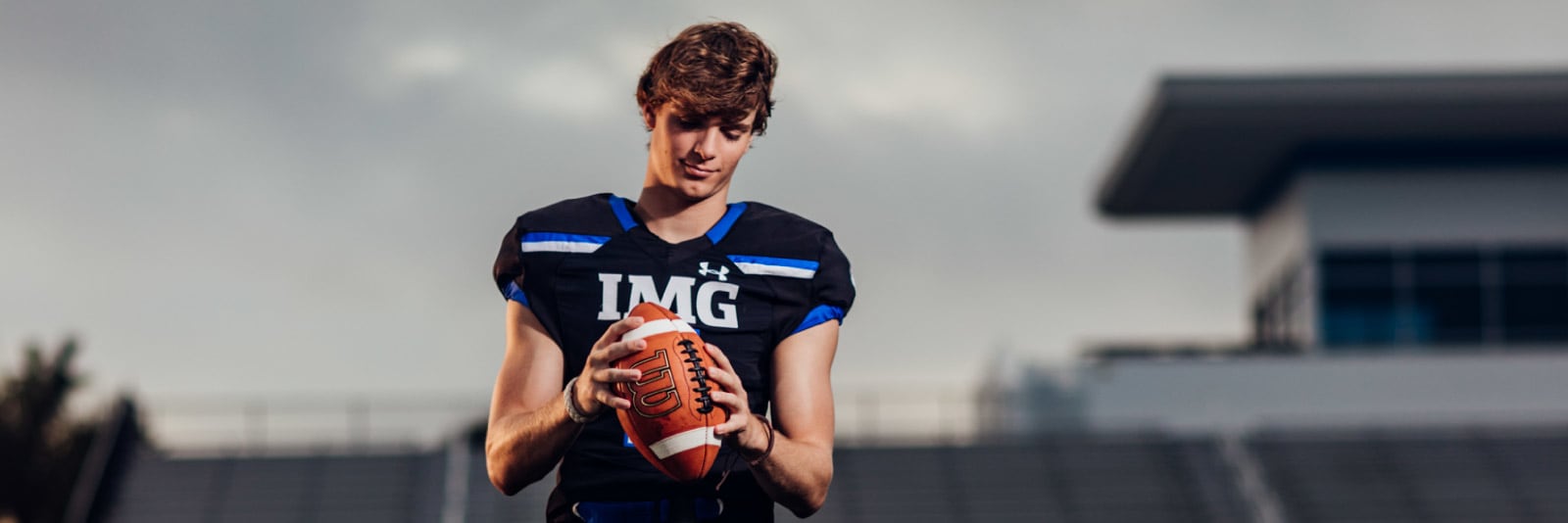The photograph is a wide, almost panoramic shot of a high school football player from the IMG Academy in Florida. The light-skinned male, who appears to be of high school age, is depicted from the waist up, wearing a black football jersey with white "IMG" lettering on the front, accompanied by blue and white stripes on the shoulders. An Under Armour logo is also visible on the jersey. The player is holding a football in front of him, looking down at it with a smirk. His longer hair frames his face, and he is sporting a bracelet on his left wrist. The backdrop reveals a blurred image of high school grandstands or bleachers, complete with a press box. A light blue sky, dotted with clouds, can be seen behind him, though the subject is illuminated as if by a flash. Overall, the setting and details suggest this is a typical high school sports photo shoot aimed at highlighting the player, potentially a quarterback, in a flattering and professional manner.